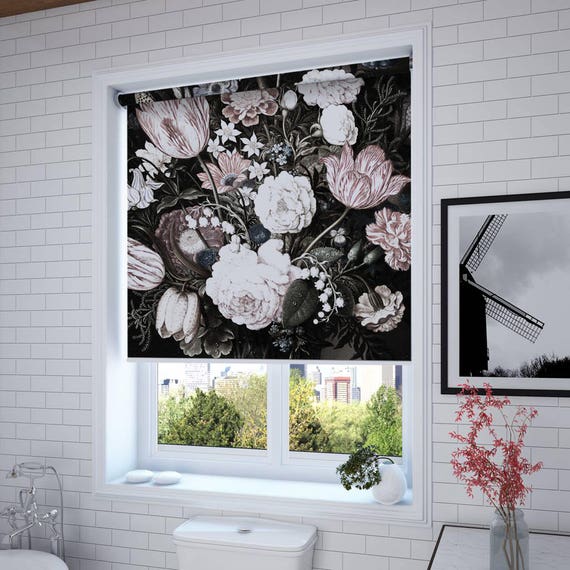The photo captures a detailed view of a bathroom interior. Dominating the space are white subway tile walls and a central rectangular, double-paned window encased in white molding. The window features a partially pulled-down roller shade with a striking black background adorned with delicate white and pink floral patterns. The upper portion of the window shows the exterior view of lush green trees, while the lower section displays two white, oval bars of soap on the left side of the windowsill and a small white vase with a green plant on the right.

Below the window sits the top of a white porcelain toilet. To the left, there's a white bathtub fitted with a silver faucet. To the right of the window, a black-framed black-and-white photo of a windmill hangs on the wall. Beneath this photo, a white marble countertop with a thin black border supports a glass vase filled with thin brown sticks and tiny red leaves. The carefully curated choice of decor elements and the blend of functional fixtures create a harmonious and aesthetically pleasing bathroom environment.